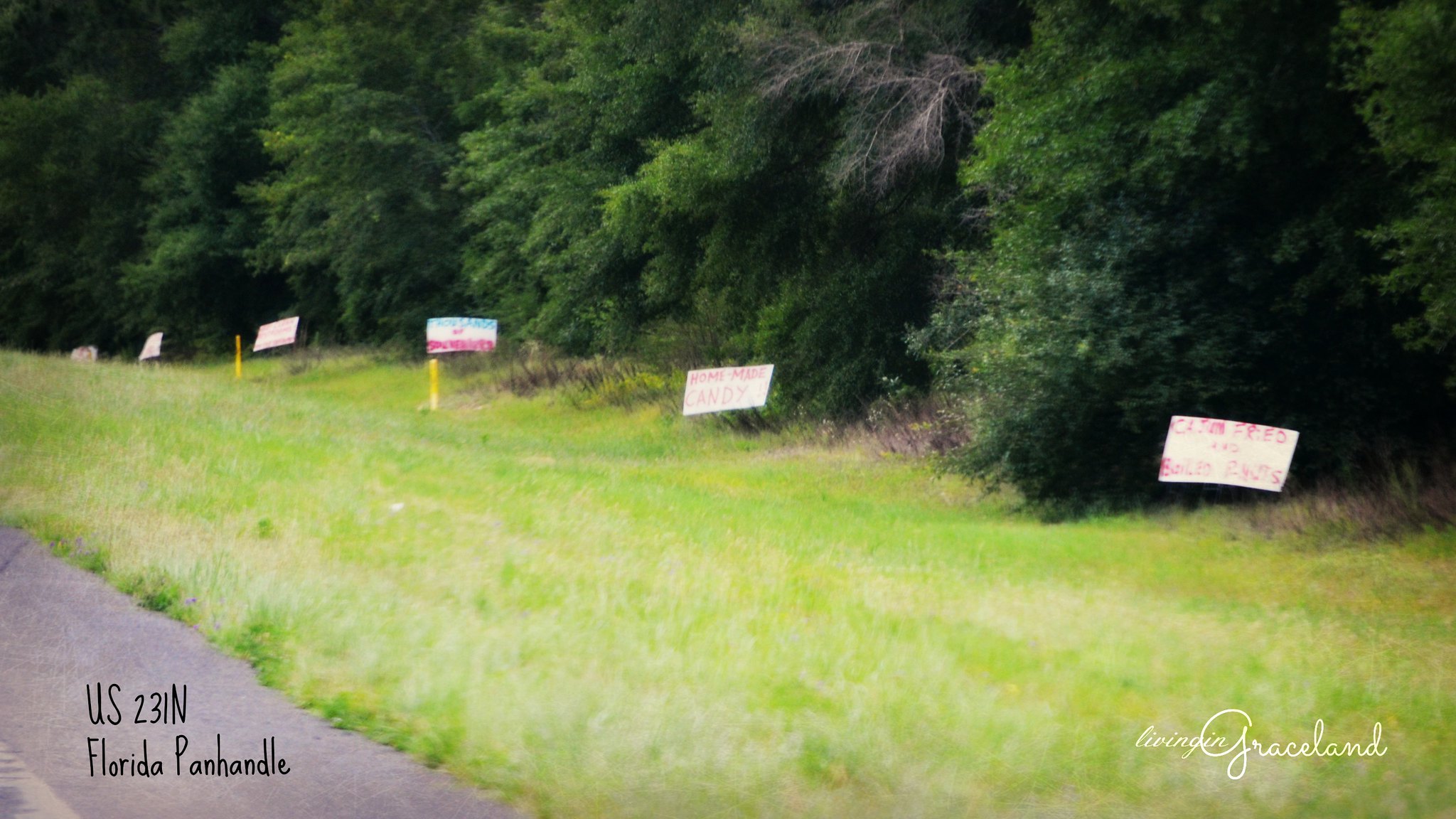In this professionally shot photograph taken on the side of a highway, several key elements draw the viewer's attention. The image includes text in both the bottom right and left corners—for instance, the bottom right corner reads "Florida Panhandle" along with a number, while the bottom left corner features the phrase "Living in Graceland" written in cursive. The setting prominently features a thick, lush forest with large, bushy green trees extending across the background, indicating a dense, verdant area.

The foreground of the photograph showcases a wide patch of grass that spans the entire bottom half of the image. Various signs, all printed on rectangular white pieces of paper, punctuate this grassy expanse. These signs are adorned with what appears to be red, handwritten lettering. Additionally, the lower left corner of the image reveals a portion of the highway's gray asphalt, providing context and further emphasizing the roadside setting.